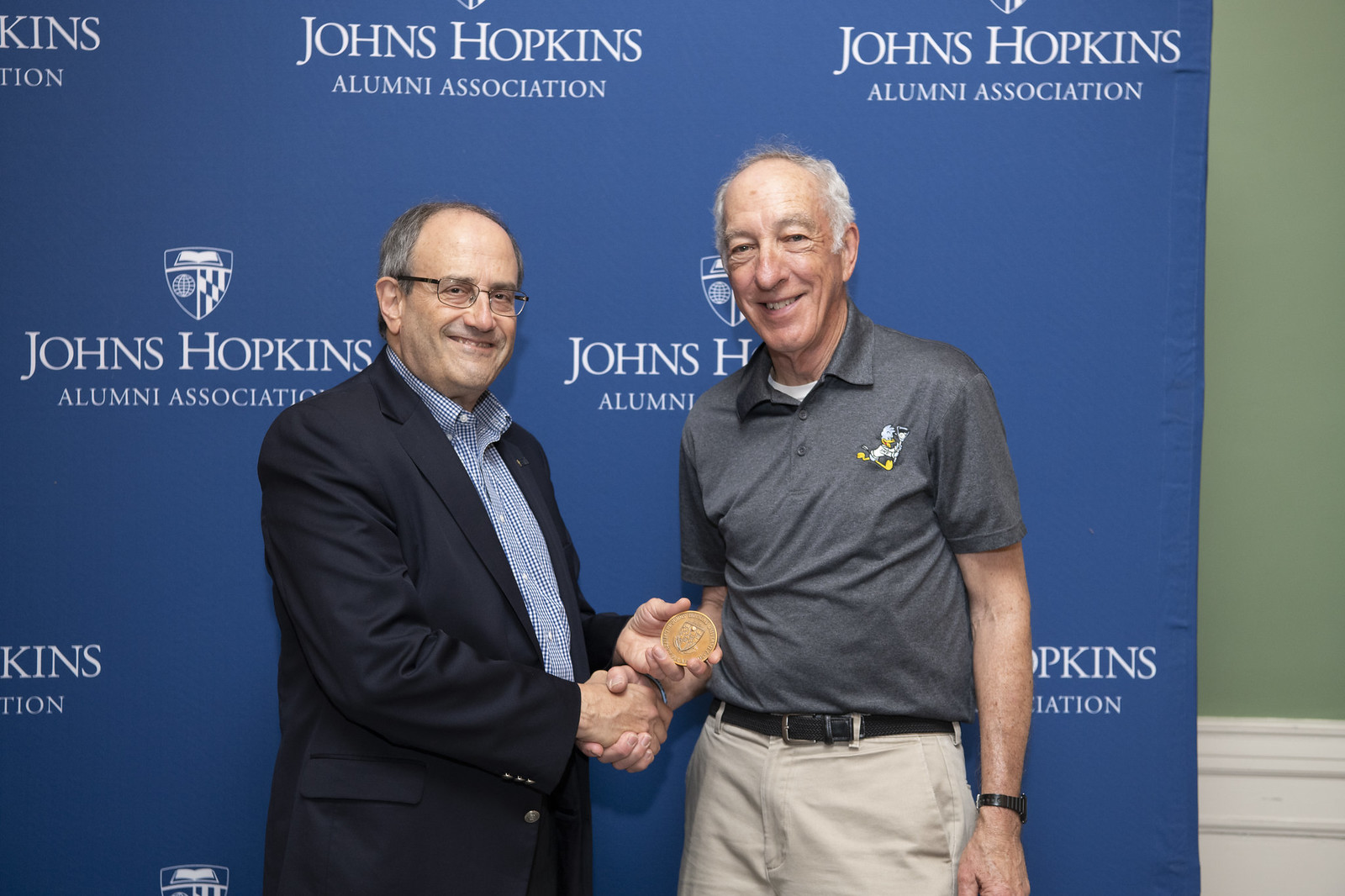In this photograph, two elderly men are standing side by side, shaking hands and smiling for the camera, set against a blue backdrop emblazoned with the "Johns Hopkins Alumni Association" logo. The man on the left, appearing to be in his 70s, is a white male with thin gray hair, glasses, and a balding head. He is dressed in a navy blue suit coat over a light blue and white small-checkered button-down shirt, and is holding a bronze-colored round medallion in his hand. The man on the right, possibly in his 80s, is also balding with gray hair, and is dressed in a gray short-sleeved polo shirt featuring a duck cartoon insignia, tan pants, and a black belt. Both men are looking forward with big smiles, suggesting a celebratory moment or an award presentation. To the far right of the image, a portion of the green wall with a white border is visible, further adding to the formal setting of the scene.